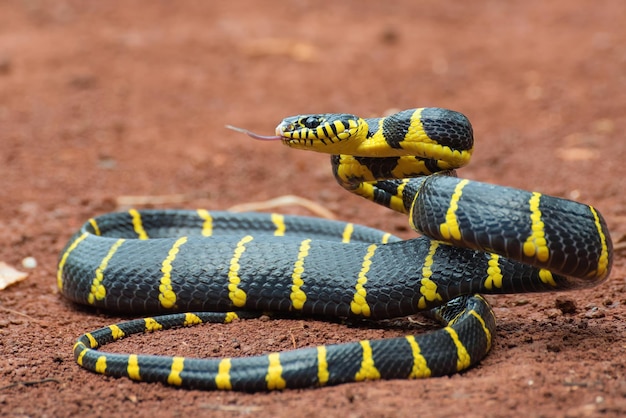This photograph, taken outdoors, centers on a striking snake coiled on a bed of reddish-brown soil. The snake, predominantly black with vivid yellow stripes running vertically along its body, appears poised to strike. Its head, which is more yellow with thin black stripes around the mouth, is facing to the left with an ominous black eye visible. The snake's tongue, a distinct pink, protrudes, heightening the impression of imminent attack. The background remains blurred, highlighting the snake’s sinuous form and textured skin, while emphasizing the snapshot's tension and intensity.